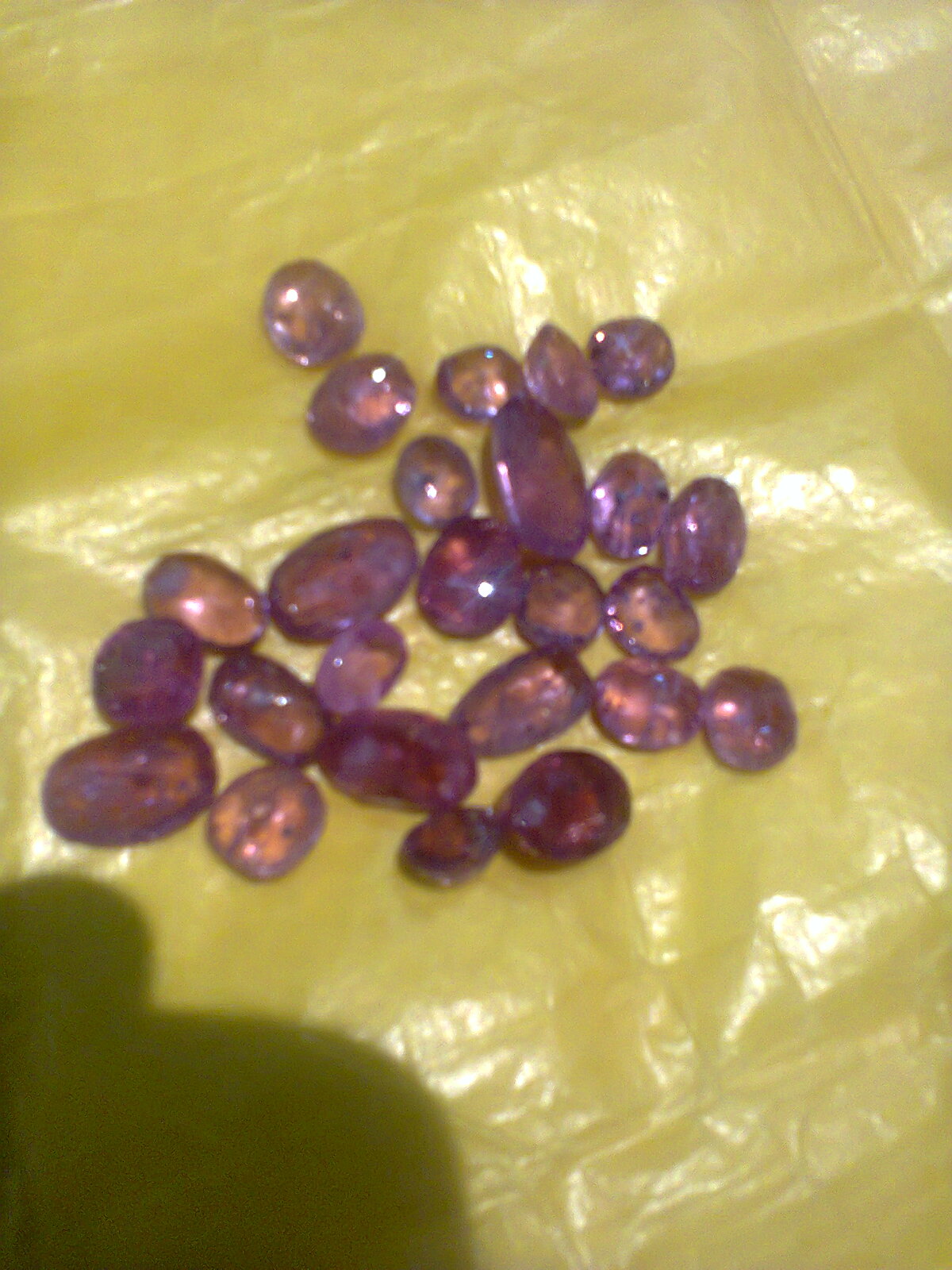This slightly blurry photograph shows a collection of approximately 20 to 25 polished amethyst stones, arranged haphazardly on a shiny yellow surface, which appears somewhat plasticky or gelatinous. The stones, varying in shape and size, range from dark purple to brown with hints of gold, and some exhibit a near-translucent quality, allowing light to pass through them. The stones and the surface beneath them both reflect the overhead light, with the stones looking particularly wet and glossy. In the lower left corner of the image, there's a shadow, likely cast by the photographer, adding an interesting element to the composition. The stones, none larger than a grape, contrast against the bright yellow backdrop, creating a vivid and eye-catching image.